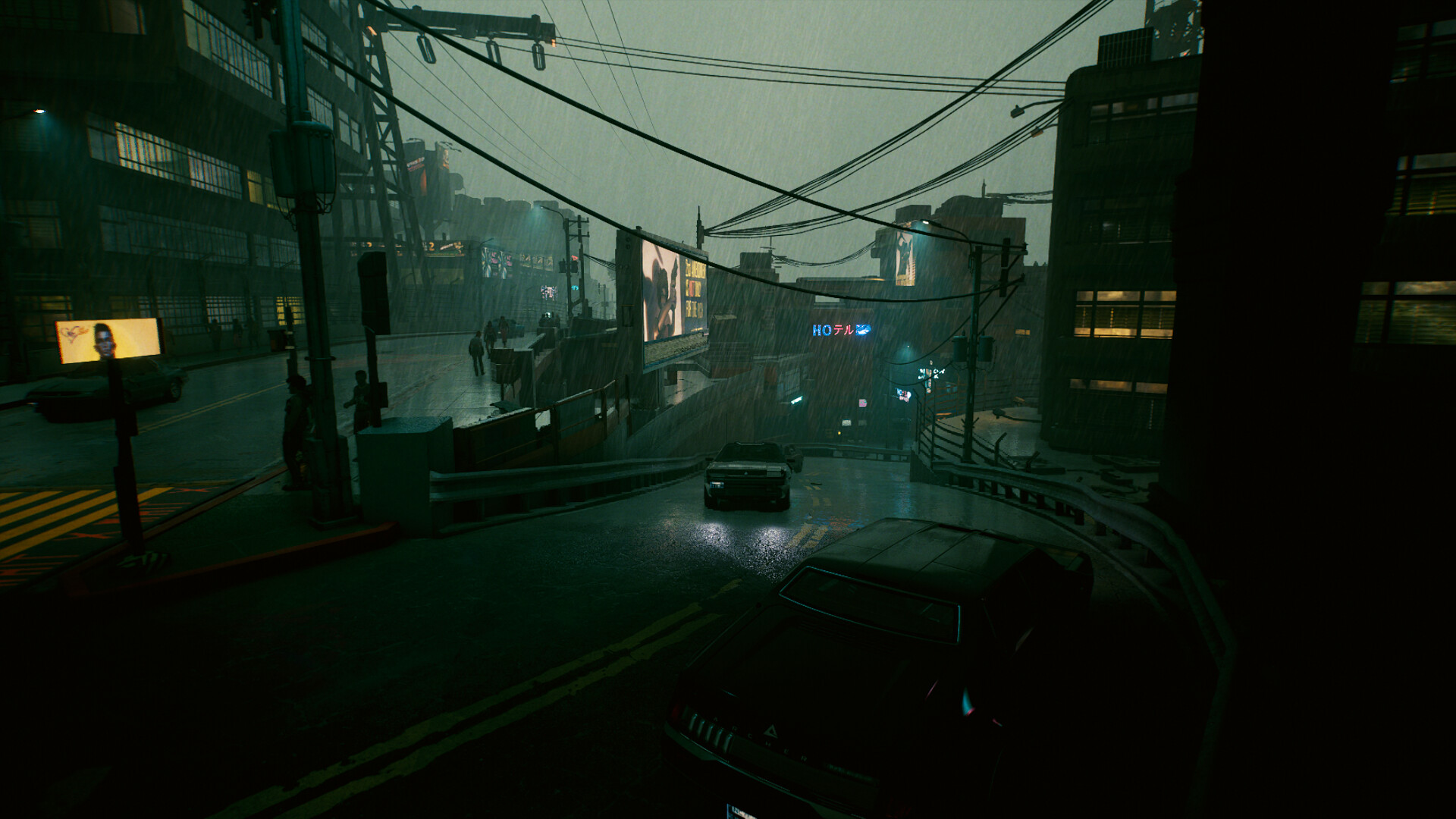The image depicts a moody, rain-soaked urban street at night, possibly from a video game scene, characterized by its twilight or overcast sky and pronounced darkness. The composition is roughly one and a half times wider than it is tall. The road forms a Y shape, splitting into two directions; the main road enters from halfway up the left side and veers off towards the 2 o'clock direction, while the other branch extends from the bottom left corner. A dark-colored car approaches from the right side of the Y. 

The scene is framed by tall, multi-story buildings, including what appears to be a commercial structure on the right and a warehouse-like building with long windows on the left, some of which emit a faint glow. The dim environment is punctuated by scattered lit windows and reflections on the wet pavement, which features distinct yellow lines, both solid and dotted. 

Overhead, numerous power lines stretch in a V-like pattern, crisscrossing the hazy, gray sky. Between the two roads, a billboard stands at an angle, its details obscured but seemingly advertising something. Further down the street, a lighted sign on a building displays the letters "HO" in blue and "FA" in red, though its full message remains unclear due to the distance and poor visibility.